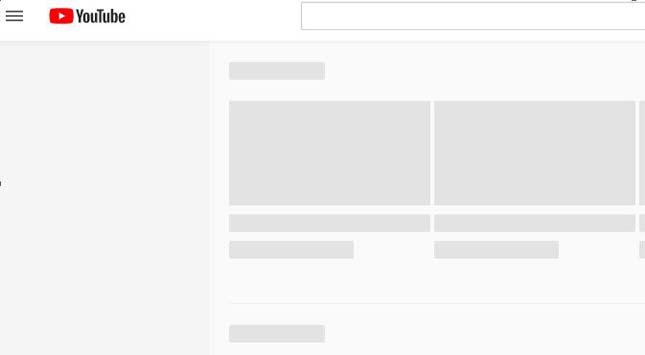The image features a minimalist interface design. In the top left corner, there are three horizontal lines, commonly representing a menu icon. Next to these lines is a red square containing a white play button symbol, indicative of the YouTube logo. To the right of the logo is a text box placeholder. The rest of the page is dominated by a monochromatic color scheme, featuring various shades of gray. The background is light gray adorned with darker gray square patterns. Centrally and prominently displayed are two large gray rectangles. Beneath each large rectangle, there is a slightly narrower gray rectangle, followed by an even thinner gray rectangle beneath that. The large rectangle on the left side has an additional narrow rectangle positioned towards its bottom, just above and below it.